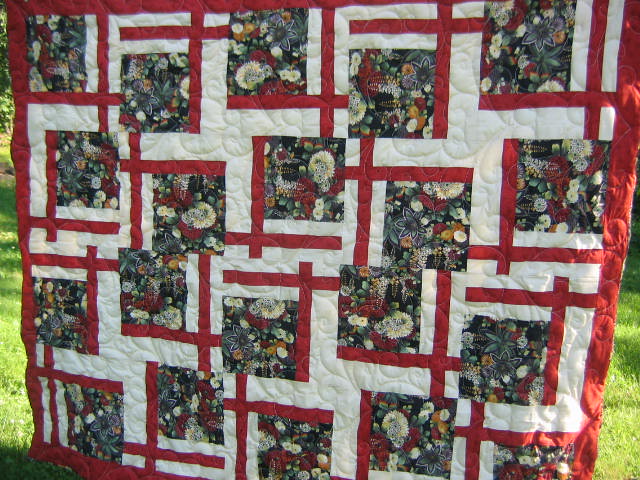This image captures a vibrant outdoor scene dominated by a hanging quilt. The backdrop features a lush, bright green lawn bathed in sunlight, with shadows hinting at a clear, sunny day. The quilt, prominently displayed in the foreground, is quite large and framed by a bold red border. It showcases an intricate pattern of red lines forming unclosed squares on a white background. Within the intersections of these lines are vivid floral patches, bursting with white, red, blue, purple, and yellow flowers, resembling asters and daisies. The fabric's floral design appears dense and lively, creating a bouquet-like effect. Additionally, the white areas of the quilt are adorned with intricate, swirling quilting patterns, adding depth and texture to the piece. The light striking the right side of the quilt enhances its rich colors and detailed craftsmanship.